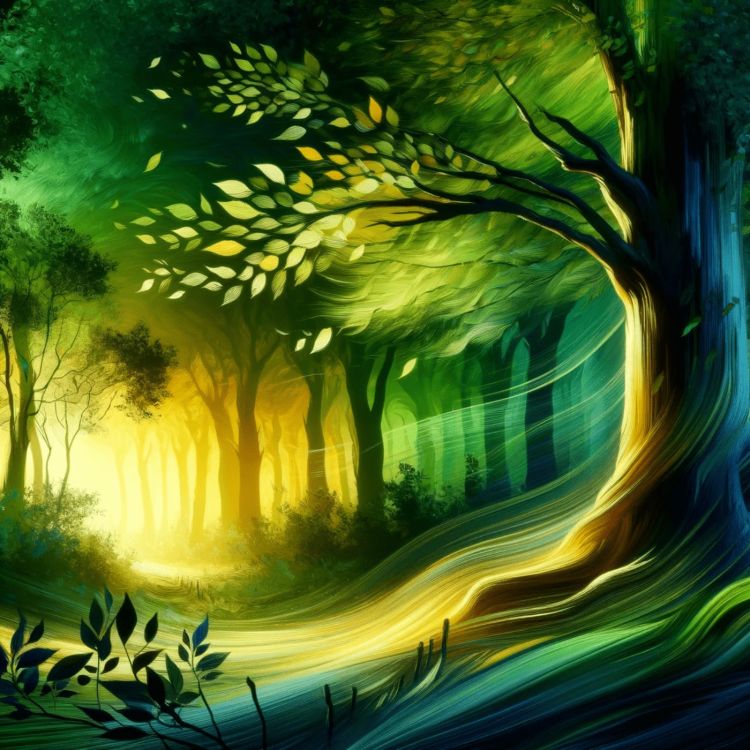This impressionistic artwork, potentially digital, depicts a forest scene on a windy night. Dominating the right side of the frame is a prominent tree trunk, from which swirls of light and color—mainly yellow, brown, and black—emanate and extend toward the forest floor on the left. The tree trunks and their dense foliage, featuring shades of green and yellow, create a textured backdrop. The swirling lines and movement suggest a strong wind, causing some leaves to appear as if they’re falling. Notably, a bright yellow light illuminates the midsection on the left, hinting at an intense light source, possibly sunlight, penetrating the dense forest. In the foreground, the forest floor shows some green leaves and plants, adding to the detailed, albeit stylized, composition.